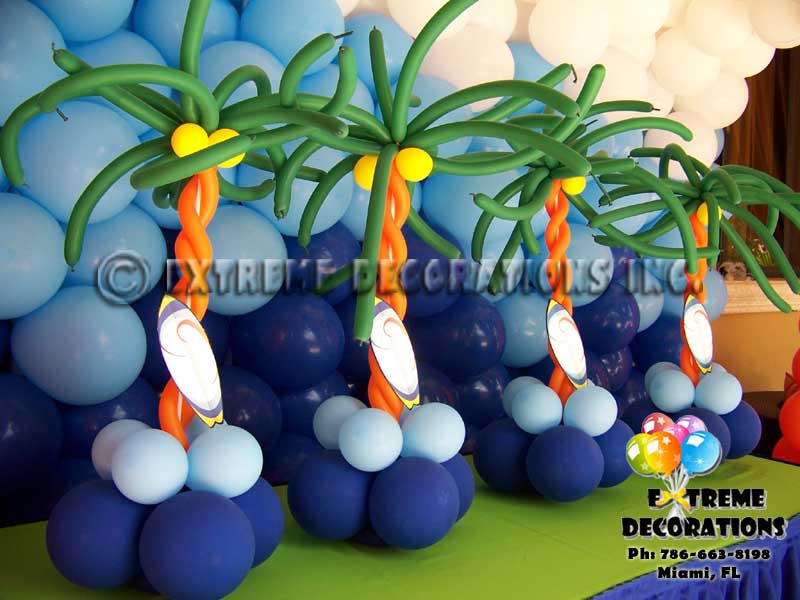This image showcases an elaborate balloon arrangement by Extreme Decorations, Inc. at a stage setup in Miami, Florida. Ornate clusters of balloons, primarily in shades of blue and white, are scattered throughout the scene. In the foreground, darker blue balloons provide a base, with lighter blue balloons layered above them. The top section of the display features twisted green balloons shaped to resemble palm tree fronds, supported by orange balloons fashioned into tree trunks using a helical twist pattern. Atop the orange balloon trunks are yellow balloons mimicking coconuts. Each of the four palm tree decorations is adorned with surfboard-like oval paper pieces leaning against them, contributing to the tropical theme. The arrangement is bordered by a green tarp on the stage, with additional white balloons in the upper right corner. A watermark reading "Extreme Decorations, Inc." and the contact number "786-663-8198, Miami, Florida" are prominently displayed on the image, indicating the company's branding and location.